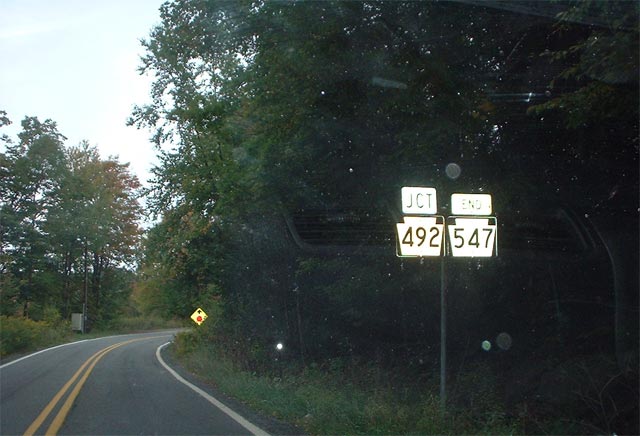This photograph captures a serene, curving roadway flanked by lush forests on both sides. The road, a single lane in each direction, is marked with a double yellow line in the center. To the right of the road, two rectangular signs are positioned, both bordered in black and inscribed with white and black text. The top sign reads "JCT 492," while the bottom sign bears the number "547." The entire scene evokes a peaceful journey through dense woodland, underlined by the detailed road signs providing direction and guidance.